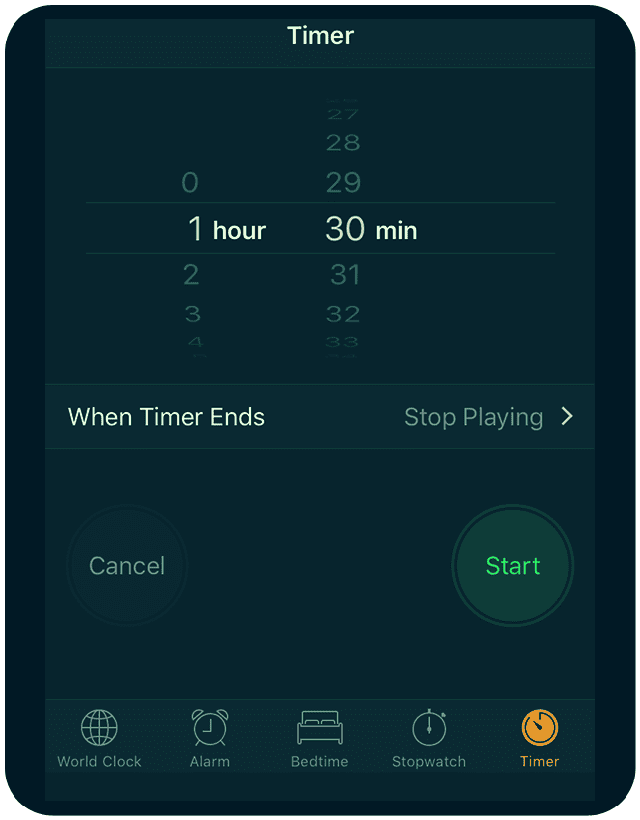This detailed and cleaned-up caption describes a screenshot from either a tablet or smartphone showing a time-setting application:

---

The screenshot displays the interface of a time-setting application on a tablet or smartphone. The background is dark blue or black, with a dark blue header banner at the top. In the center of this banner, the word "Timer" is written in a faded white with a subtle blue tint. Below the header, against a darker blue backdrop, there is a cascading display of numbers forming a 3D-like arc, used to set hours and minutes.

On the left side, the numbers represent hours. The '1' is highlighted in white, indicating it is selected, with the word 'Hour' beside it. The numbers '0', '2', '3', '4', and a partial '5' curve around it.

On the right side, the numbers represent minutes. The '30' is highlighted in white, indicating it is selected, with the acronym 'MIN' for minutes beside it. The numbers '26', '27', '28', '29', '31', '32', '33', and the start of '34' are also visible in blue.

Below these numbers, there is a floating rectangle with a light blue border containing two sections of text. On the left, in white, it says "When Timer Ends" with leading capitals (W, T, E). On the right, in blue, it says "Stop Playing" with capitals (S, P), accompanied by a white right-pointing arrow.

At the bottom of the screen, there are two buttons. The left button is blue with cyan-blue text that reads 'Cancel'. The right button is green with forest or neon green text that reads 'Start'.

On the bottom bezel, there are icons for different features of the application arranged in a row:
1. A globe icon labeled 'World Clock'.
2. An old-style alarm clock icon labeled 'Alarm'.
3. A bed icon labeled 'Bedtime'.
4. A stopwatch icon labeled 'Stopwatch'.
5. An orange and blue kitchen timer icon labeled 'Timer', which is selected and displayed with orange text instead of blue.

---

This thorough description efficiently captures all relevant details seen in the screenshot.